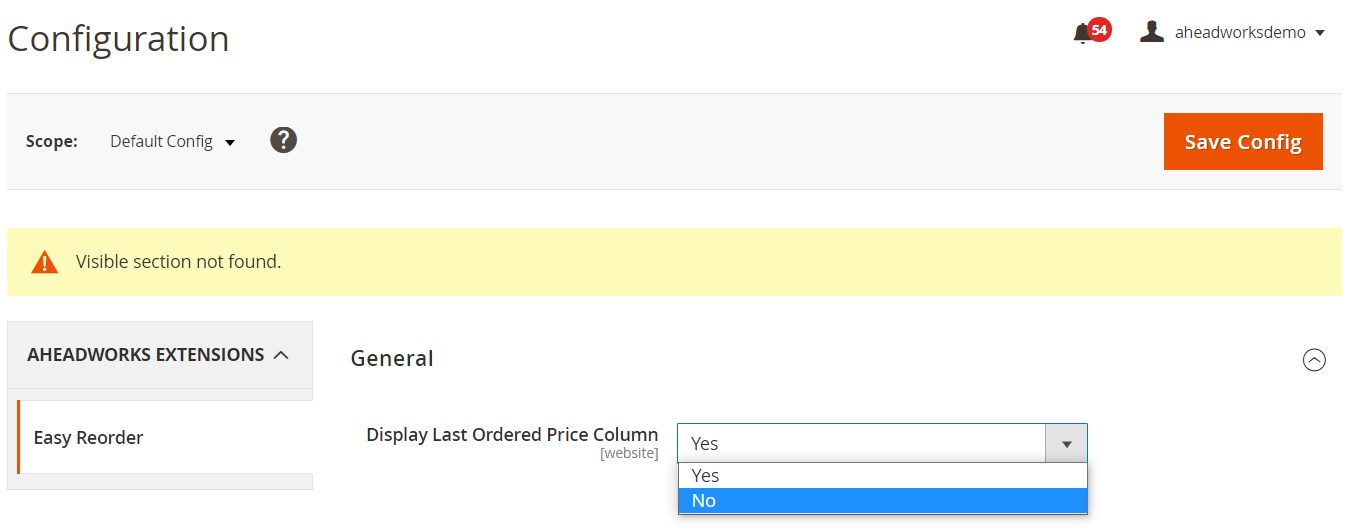The screenshot displays a webpage interface focused on configuration settings for an application. In the top left corner, the heading "Configuration" is prominently visible. At the top right of the screen, there's a bell icon with a red notification badge displaying the number '54', indicating pending notifications. Next to the bell icon, a person icon is labeled "Ahead Works Demo" with a downward-pointing arrow, suggesting a drop-down menu for user options.

Directly below the "Configuration" heading, the word "Scope" appears, followed by a drop-down menu set to "Default Config". Nearby, a small circle houses a white question mark, likely symbolizing a help or information section.

Beneath the user icon labeled "Ahead Works Demo", there is a prominent orange button that reads "Save Config". Underneath this button, a large yellow banner spans across the screen, containing a red triangle with a white exclamation mark and the message "Visible section not found".

Below the yellow banner, another menu is visible. It lists "Ahead Works Extension" and "General" with an upward-pointing arrow to the far right. Under the "Ahead Works Extension" section, there is a text box labeled "Easy Reorder", and the option "Display Last Ordered Price Column" is visible with a drop-down menu currently hovering over "No". The entire webpage has a clean white background with no additional text or elements.